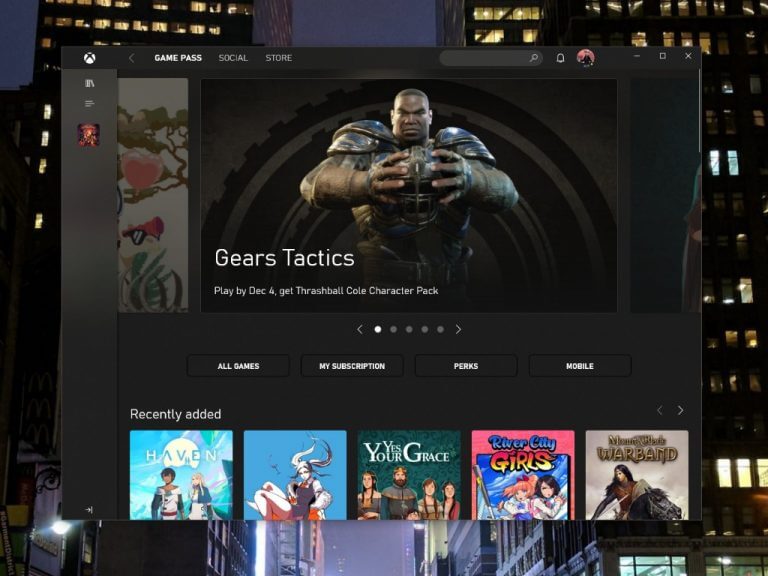A screenshot captures the interface of a gaming platform, predominantly featuring a dark color scheme with a black and gray aesthetic. The perimeter of the screen displays high-rise buildings at night, emphasizing illuminated windows against a predominantly black backdrop. Central to the interface is a horizontally rectangular section. 

In the upper left corner of this main section, navigation tabs labeled 'Game Pass,' 'Social,' and 'Store' are present, resembling a familiar layout akin to streaming services like Amazon Video. The showcased game in this section is "Gears Tactics," depicted through a prominent image of an armored football player—a black man holding a helmet and exuding a stern demeanor. Accompanying this visual are white text labels that read: "Gears Tactics" and "Play by December 4th, get Fresh Ball Cold Character Pack."

Below the featured game are a series of slider dots indicating a carousel menu, facilitating navigation through various screens. Beneath the slider dots, four buttons appear from left to right, labeled 'All Games,' 'My Subscription,' 'Perks,' and 'Mobile,' outlined in black against a dark gray background.

At the bottom of the interface, there is a row of five thumbnails representing recently added games. The games featured include "Raven," another with a cartoon image but no visible name, "Yes, Your Grace," "River City Girls," and a partially obscured title, presumably "Warband." The overall design suggests a user-friendly gaming hub that enables easy navigation and selection of various game titles and features.